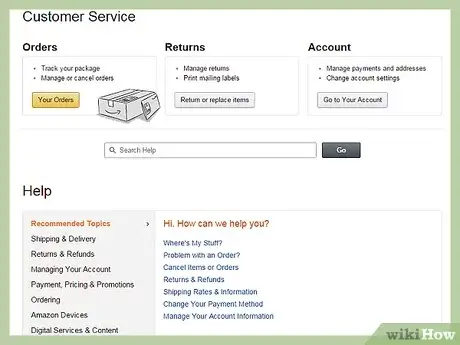The screenshot features an online customer service interface set against a white background. Prominently displayed are various options for managing orders and account settings. At the top, a bright orange rectangle labeled "Your Orders" allows users to track packages, manage, or cancel orders. Within this section, there are further options to "Returns," "Manage Returns," and "Print Mailing Labels," all accompanied by a gray rectangle titled "Return or Replace Items."

Under "Account Management," users can manage payments and addresses or change account settings, with a directed gray rectangle labeled "Go to Your Account." At the top of the interface is a search bar featuring a magnifying glass icon on the left and a gray rectangle with the word "Go" in white.

To the right, a help section beckons with "Hi, how can we help you?" inquiring about queries. Underneath, blue text links offer visitors quick access to solutions for "Where's My Stuff," "Problem with an Order," "Cancel Items or Orders," "Returns and Refunds," "Shipping Rates and Information," "Change Your Payment Method," and "Manage Your Account Information."

At the bottom of the page, a green rectangle directs users to "Wikia How," suggesting an additional resource for assistance.